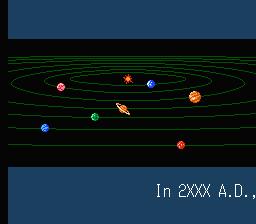This is a highly detailed digital rendering of the solar system, centered within a black horizontal rectangle reminiscent of a widescreen movie format. The Sun, depicted as an orange starburst, anchors the center of the image with faint green lines outlining the orbits of the eight planets. The background primarily features a deep black with blue rectangular bars above and below the solar system for added contrast.

Starting from the left of the Sun, we observe a mix of planets: three to the left and four to the right. Earth is to the right of the Sun, followed by Jupiter. Saturn, distinctly recognizable by its tilt and vibrant yellow rings, is positioned lower center, extending towards the right. A red planet, likely Mars, is also prominently displayed to the right. Further to the left, a pink planet bordered in white, and a blue planet are visible. There's also another blue planet to the right of Saturn, and a green planet in its vicinity. Additionally, Pluto is situated at the far lower right, and a fiery depiction suggests either a planet with an intense illumination or a meteor.

Details that stand out include the background's blackness, accentuated by medium blue rectangles framing the screen's upper and lower parts. A thin vertical black line marks the left side. In the bottom right corner of the screen, white text reads "IN2XXXAD," suggesting some form of identification or timestamp for this computer-generated rendering. The overall scene showcases a meticulously crafted and vividly colored representation of our solar system, with each planet illustrated in a unique hue and the entire arrangement evoking a sense of cosmic intrigue.